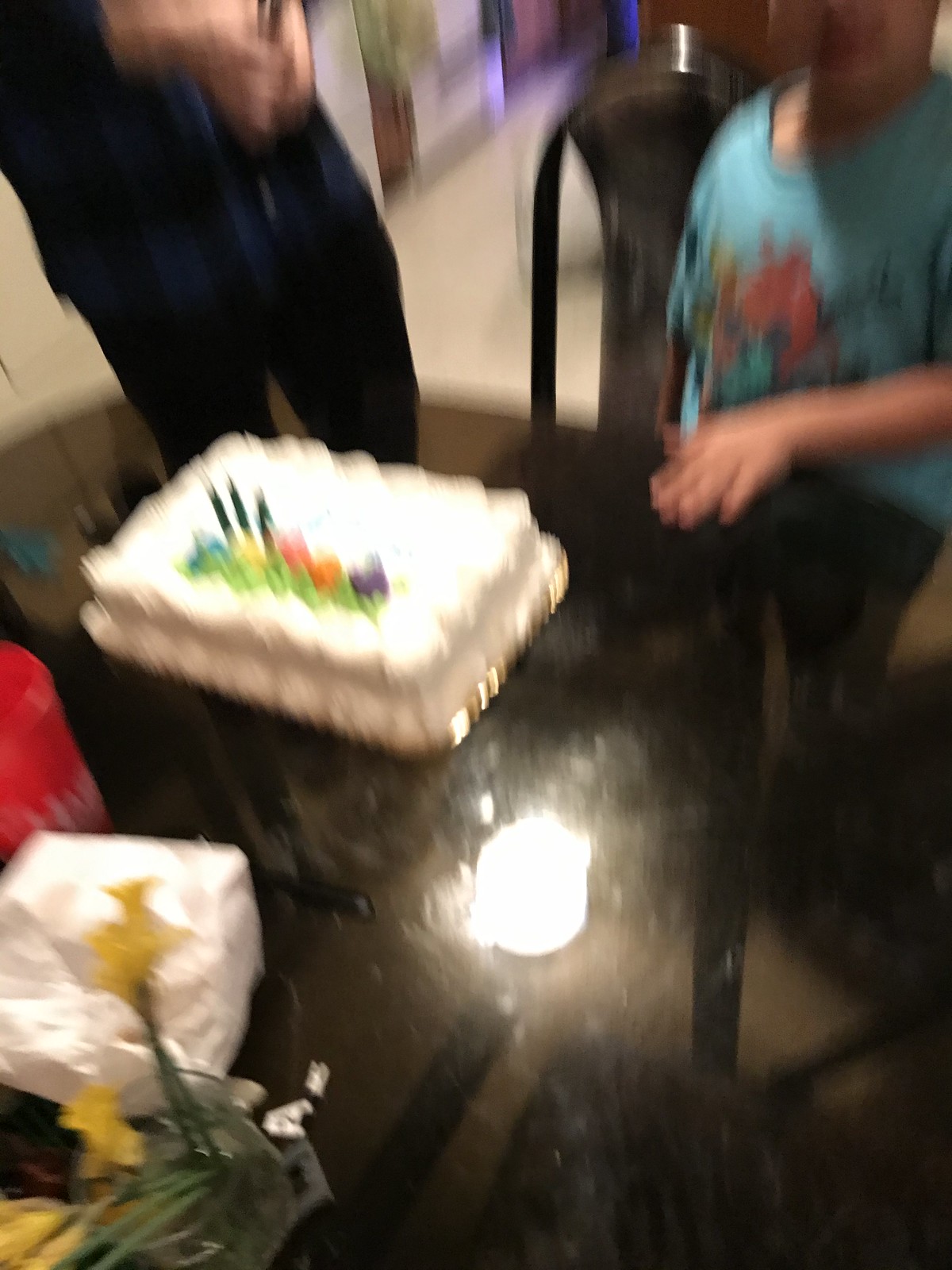The somewhat blurry image depicts an oval-shaped, dark-colored, possibly black table. On the upper right-hand side of the table, there's a small child with fair skin and wearing a light blue t-shirt adorned with graphic designs in red and green. The child, appearing to be around three years old, has their left hand raised. Adjacent to the child is a black chair. In the upper left-hand corner of the image, the lower half of an adult wearing all black is visible, with their hands blurred together. On the table rests a rectangular white sheet cake with birthday decorations, including three candles, indicating the child's age. The cake is adorned with colorful elements in orange, green, pink, yellow, and blue, though the details are indistinct due to the blurry nature of the photograph.